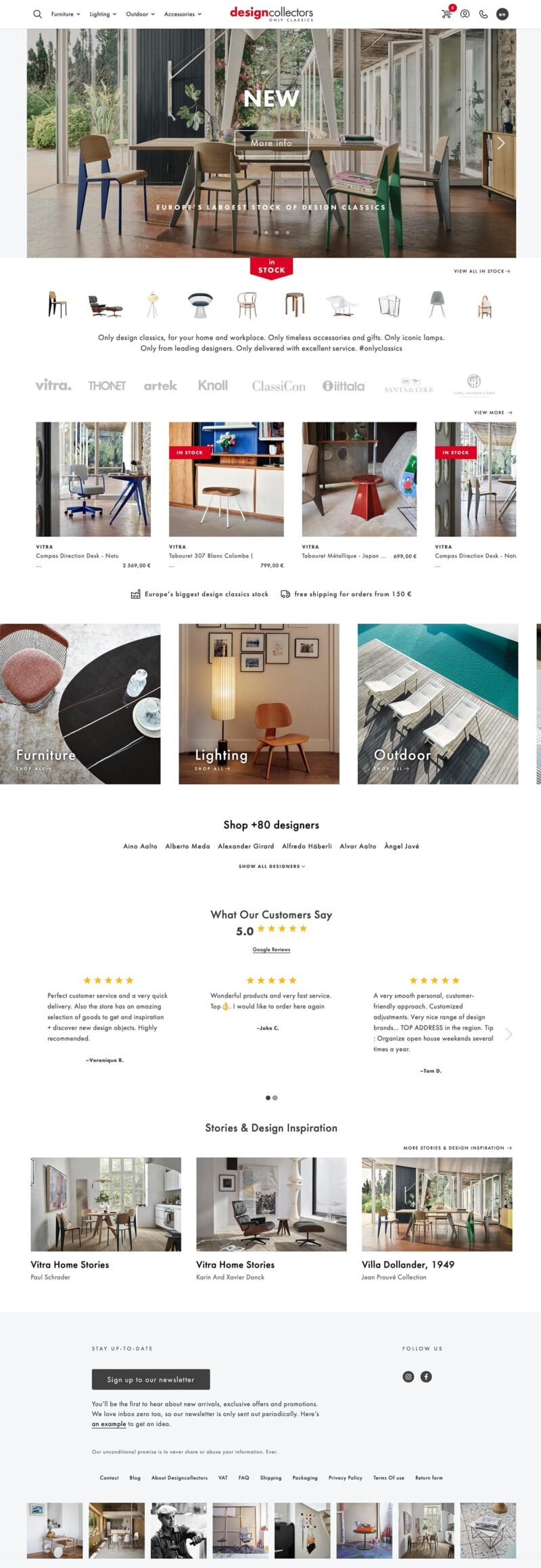Screenshot Description: Design Collector Website Overview

This image is a detailed screenshot of the Design Collector website. The website has a vast layout, indicating it is a comprehensive online store. Due to the small size of the text, the screenshot required zooming in for clarity.

At a zoom level of 121%, the top section features the website's name, "Design Collectors," centrally positioned. Below, a navigation menu with categories such as "Furniture," "Lighting," "Cushion," and "Accessories" is visible. On the right side of this menu are the "Cart" and "Contact" buttons.

Beneath the navigation bar, there is a main image showcasing a wooden table with surrounding chairs, windows in the background, and doors with the label "NEW" in the center. A "More Info" button is also present. A headline reads, "Europe's Largest Stock of Design Classics In Stock."

Further down, the website highlights various categories with images of chairs and tables. Captions include "Only Design Classics for Your Home and Workspace," "Only Timeless Accessories and Gifts," "Only Classic Lamps," "Only from Leading Designers," "Only Delivered Excellent Service," and "#OnlyClassics."

A brands section lists names like Vitra, Thonet, Architect, Knoll, Classic Co, Con, and Atelier, though some brand names were illegible.

The site also features images of specific product types:
- A pink chair on a brown rug labeled "Furniture"
- A tall floor lamp next to a wooden chair with wall art labeled "Lighting"
- Lounge chairs near a swimming pool labeled "Outdoor"

The footer encourages visitors to "Shop +80 Designers" and includes a section for customer reviews, displaying three five-star ratings. It also has a segment titled "Stories and Design Inspiration," with three images depicting well-furnished rooms. Titles under these images include "Vitra Home Stories" and "Villa de Lander 1949."

At the bottom, there is a newsletter sign-up section accompanied by seven more images showcasing various designer products.